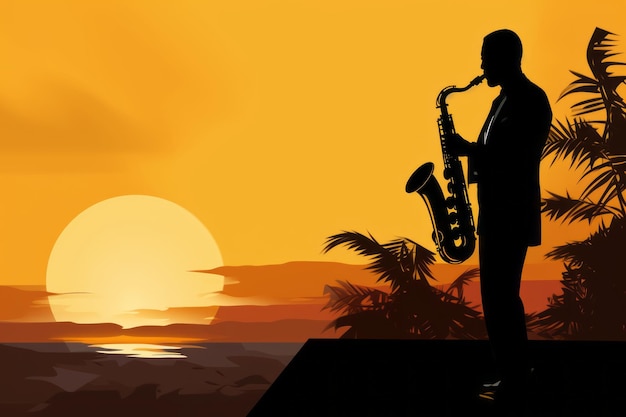The image depicts a serene sunset over a vast expanse of water, with the sun partially dipping below the horizon, casting a stunning gradient of colors that transitions from lightish yellow to deep brown. The sky is adorned with a few low-hanging clouds that catch the fading light in shades of orange. In the foreground, a man silhouetted in black stands atop a cliff or platform, exuding a calm, reflective mood as he plays a saxophone. He is dressed casually, possibly in a coat and pants or a suit, and is surrounded by the delicate fronds of palm trees, which are also silhouetted against the vibrant backdrop. The scene is artfully stylized with posterized colors, emphasizing the mellow and tranquil atmosphere as the day comes to a close.